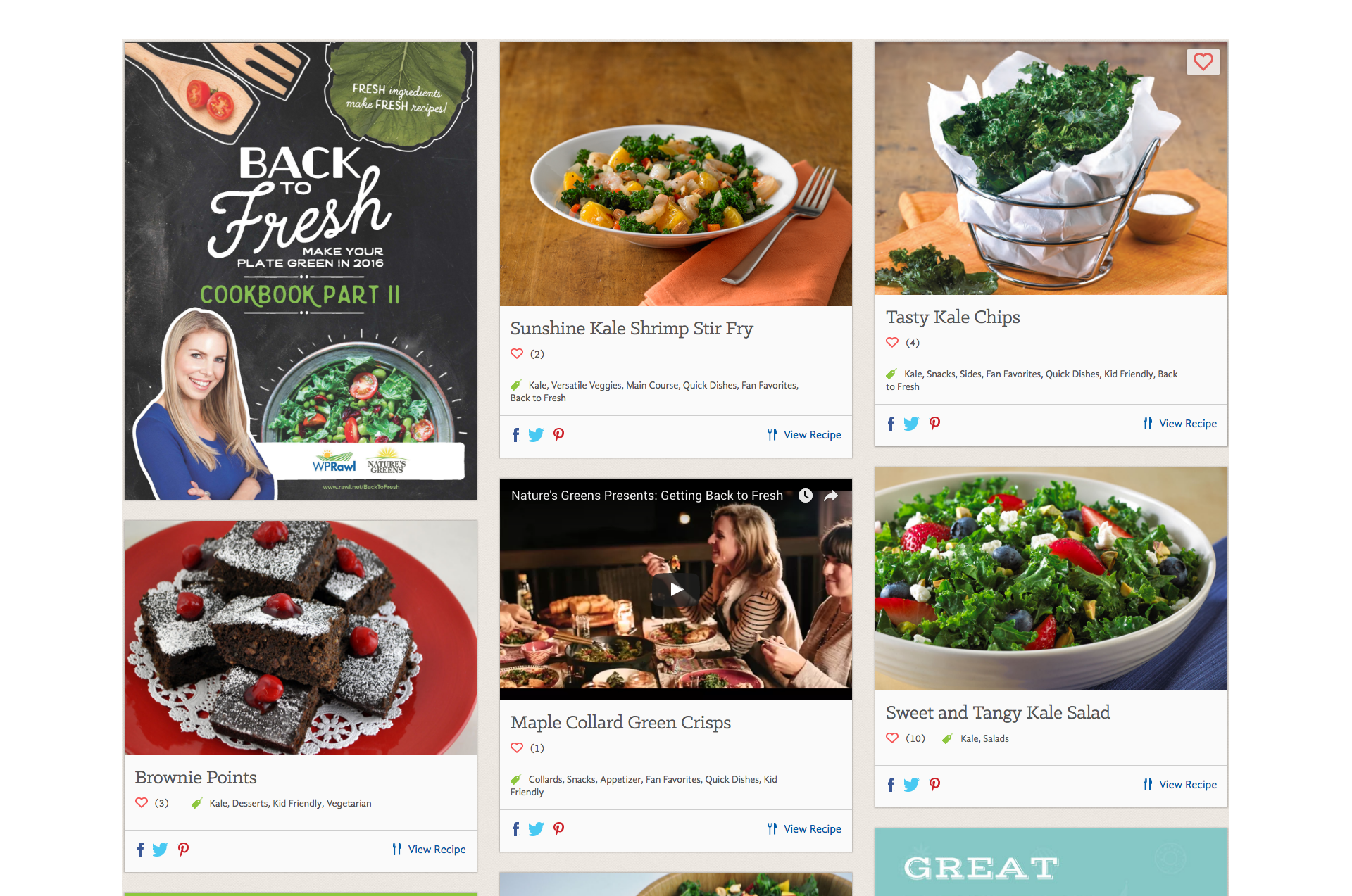**Website Food Image Gallery**

1. **"Back to Fresh: Make Your Plate Green in 2016 Cookbook Part 2"**: The upper left-hand image features a woman in a blue shirt, arms crossed, visible from the chest up. Below her is a bowl of fresh salad. The top left corner contains a wooden fork and spoon adorned with a couple of cherry tomatoes. A green leaf is positioned in the upper right corner of the image.

2. **"Sunshine Kale Shrimp Stir Fry"**: Adjacent to the first image, this photo displays a white bowl filled with a vibrant shrimp stir fry, placed on an orange napkin accompanied by a fork.

3. **"Tasty Kale Chips"**: Next, we see a metal basket lined with cloth, labeled as containing tasty kale chips. The contents look like fresh kale rather than actual chips.

4. **"Brownie Points"**: Further along, an image showcases decadent brownies topped with cherries.

5. **"Maple Collard Green Crisps"**: Following the brownie image is a dish of maple-flavored collard green crisps.

6. **"Sweet and Tangy Kale Salad"**: The final image in the series presents a beautifully arranged sweet and tangy kale salad.